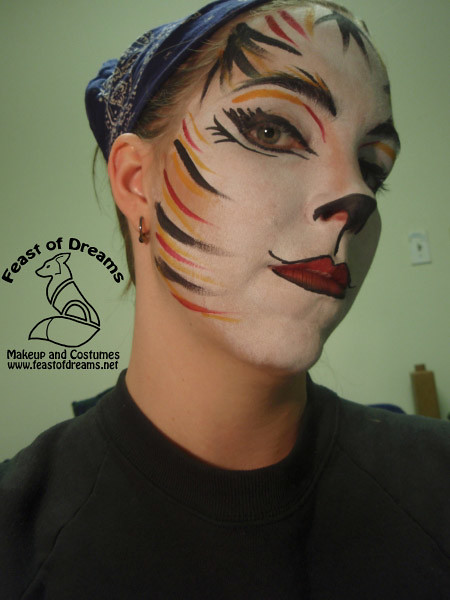In this close-up image, the young woman has skillfully applied makeup to transform herself into a cat, reminiscent of a tiger. Her face is primarily painted white, with an intricate pattern of black, red, yellow, and orange stripes circling her forehead and jawline. These stripes, varied in color and arranged in a sequence, enhance her feline appearance. She has meticulously outlined her bottom nose in black to mimic a cat's nose and adorned her lips with red lipstick, edged with black. Her eye makeup further accentuates the cat-like transformation. She wears a black shirt and has her hair tucked under a blue bandana. She also sports a silver earring. 

Behind her, the background is green with a light switch visible and turned on. A brown object is faintly noticeable in the background as well. To the left of her head, a logo featuring a fox is displayed, accompanied by the text "Feast of Dreams" above and "Makeup and Costumes, FeastofDreams.net" below, providing clear context to her makeup and costume theme. The attention to detail in her makeup and costume suggests she is prepared for a theatrical performance or a similar event.